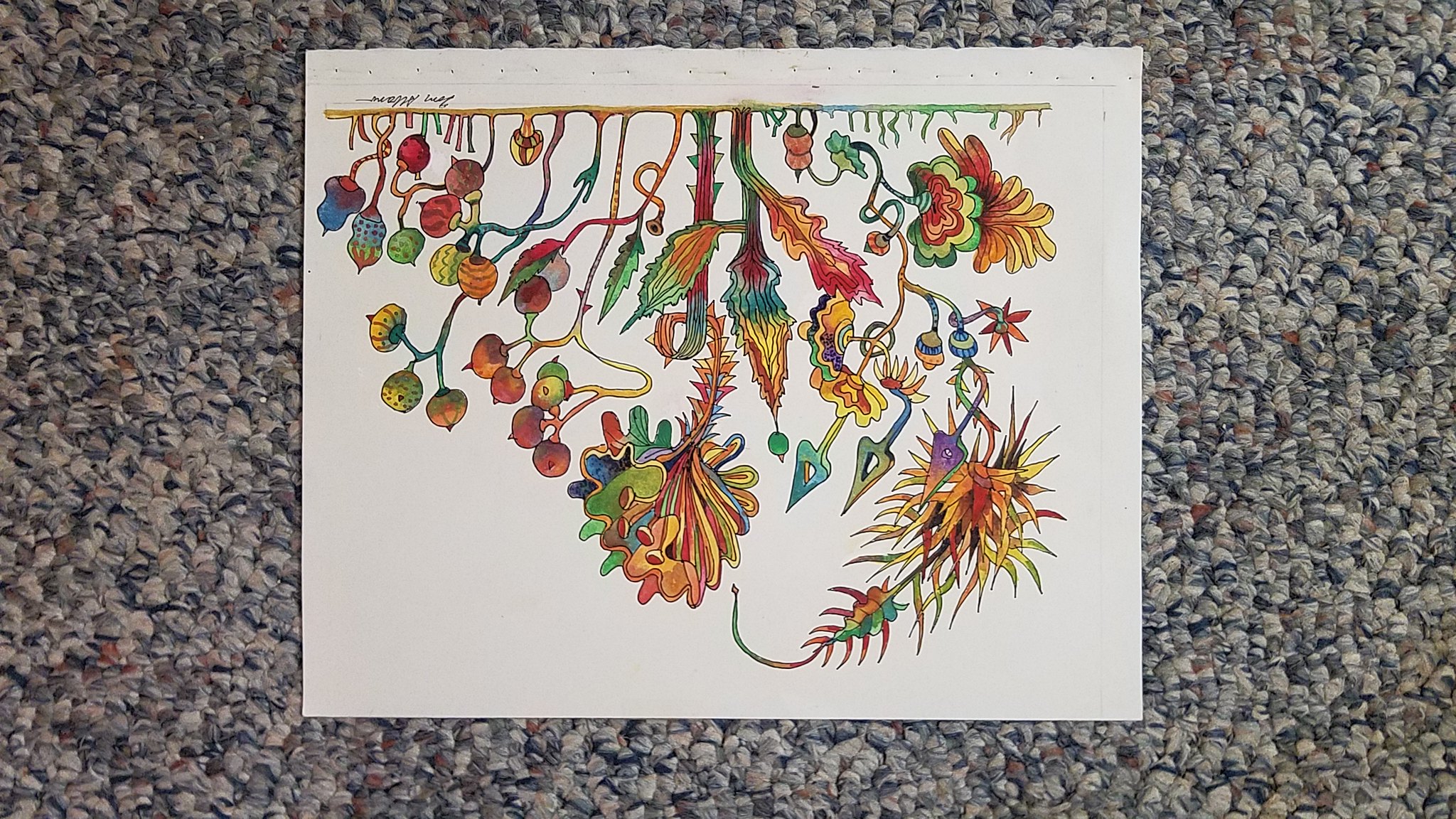This photograph captures a detailed drawing positioned centrally within a rectangular frame. The image showcases a rectangular piece of paper placed on a short-knobbed carpet, which features a mosaic of colors including white, light blue, dark blue, brown, and tan. The paper, oriented with its longer sides at the top and bottom, has a binder with multiple small holes in pairs along its top edge. The drawing itself depicts an intricate collection of plants and foliage emerging from a line just beneath the perforated edge. The botanical elements include a variety of acorns, nuts, and ferns, each meticulously illustrated to convey a sense of natural diversity and texture.